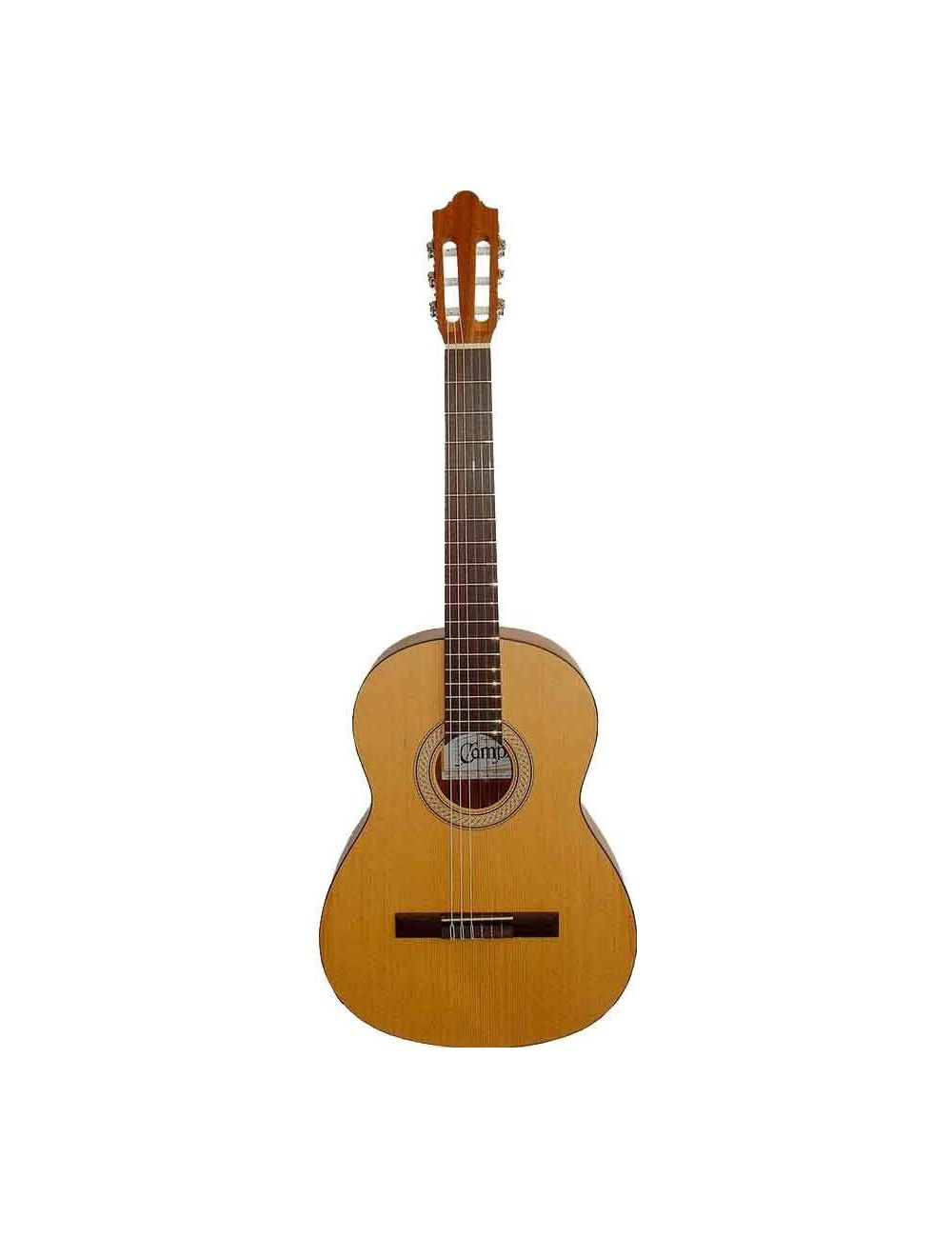This image showcases a detailed rendition of an acoustic guitar, either a high-resolution photograph or an impressively realistic illustration. The guitar, which appears to be suspended in midair against a stark white background, gives it a versatile, clip-art-like quality. The entire scene eliminates any flooring or other background elements, focusing solely on the instrument. 

The guitar features a standard design with six clear strings extending over a circular sound hole, which helps in creating reverberations. The body of the guitar is made of light blonde wood on the front, and darker brown wood on the sides and back. The neck, or strut, is similarly wooden and brown, with the headstock hosting three tuning keys crafted from reddish wood. 

Visible through the sound hole is a white label inside the guitar, displaying partial text that reads "Komp" or "Kamp," hinting at the brand. The instrument is described as being of regular size, with an overall appealing and traditional wooden aesthetic.